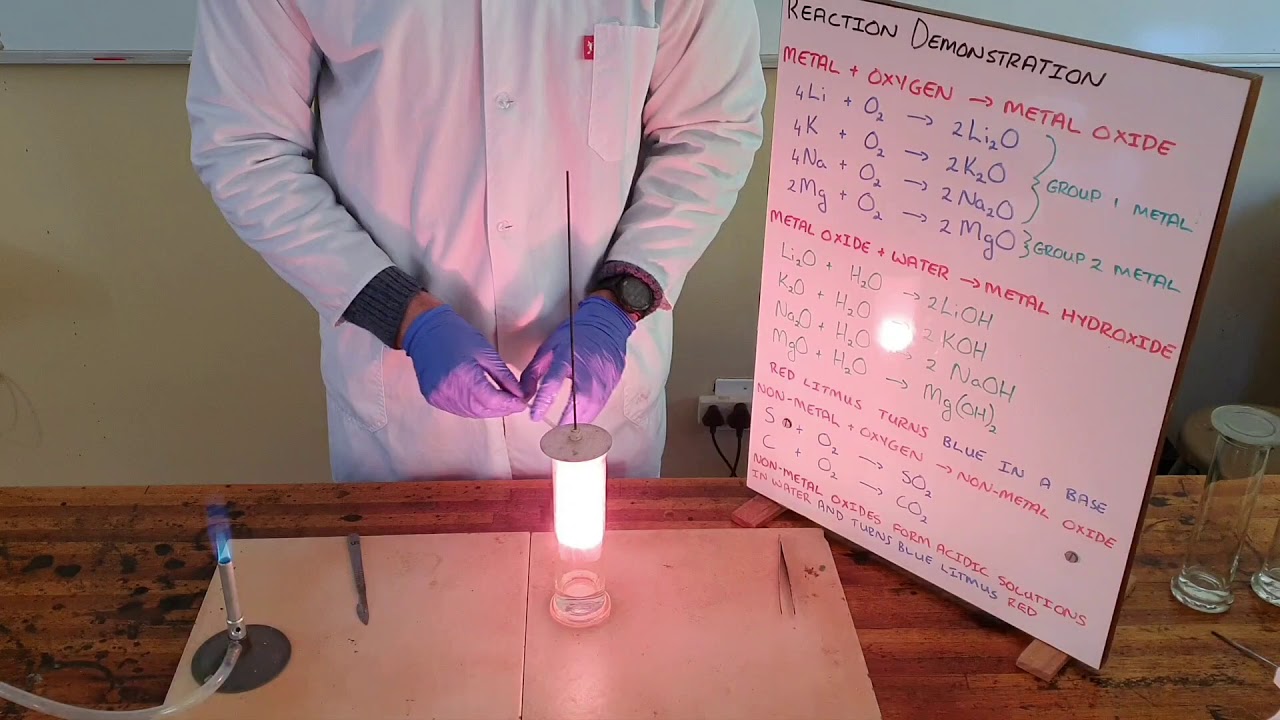In this detailed color photo of a scientific demonstration, we see the torso of what appears to be a male scientist clad in a white lab coat adorned with a red tag near the left breast pocket. He wears blue latex gloves and a black watch on his right wrist. The setting is a lab, with the scientist standing behind a brown wooden table that holds various tools and equipment. On the table lies a white mat with a pair of tweezers on the right side and a glowing tube light hanging from the ceiling, casting a white glow.

To the right on the table, there's a Bunsen burner with a visible blue flame, and a hose leading off to the left for the fuel source. Additionally, there's a lantern-like light positioned on the table, further illuminating the workspace. 

Above the table, there is a prominently displayed whiteboard at an angle that faces the viewer. The whiteboard heading reads "reaction demonstration" in black, followed by a series of chemical reactions and symbols. In red, it instructs "metal plus oxygen" with an arrow pointing to "metal oxide," accompanied by the chemical formulas for reactions involving Lithium, Potassium, Sodium, and Magnesium written in blue. Notable green squiggly lines demarcate the "Group 1 metal" and "Group 2 metal" reactions. Further down, in red, the equation "metal oxide plus water equals metal hydroxide" is displayed, trailed by more writing that becomes increasingly difficult to decipher. A clear reflection of the tube light can be seen on the whiteboard, adding to the detailed ambiance of this scientific scene.